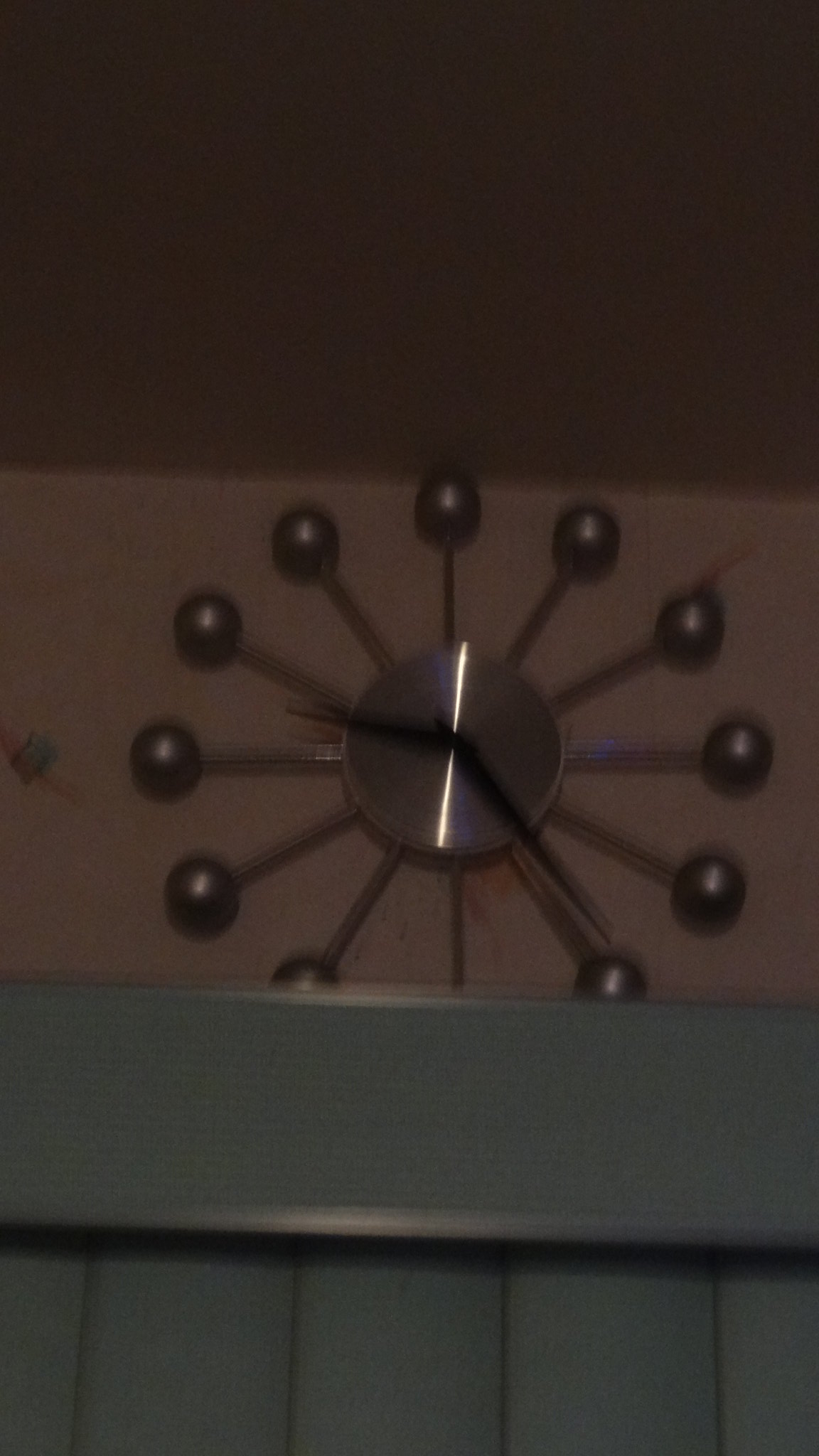A striking vertical photograph captures a unique perspective of a retro-inspired, modern wall clock. Shot from a lower angle, the image is oriented upward to highlight the clock mounted on a beige wall. The clock, resembling mid-20th century design aesthetics, eschews traditional numbers for a minimalist approach. Its central brass or metallic hub features 12 slender rods extending outward like sun rays. Each rod is capped with a small metallic ball, creating a sunburst effect. The black hour and minute hands prominently indicate a time of approximately 9:25. Below the clock, a hint of green suggests the presence of a countertop or surface, adding a subtle contrast to the beige backdrop. The overall composition, with its clean lines and evocative design, captures the blend of nostalgia and modernity in this decorative timepiece.